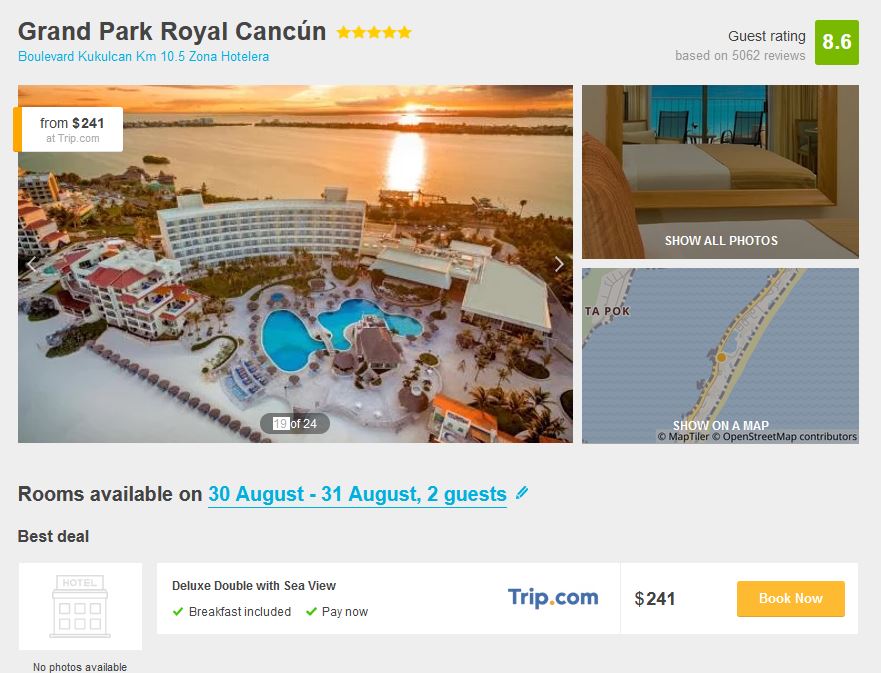The advertisement showcases a luxurious offer for the Grand Park Royal Cancun. At the top, a gray square features the name "Grand Park Royal Cancun" in black text in the upper left corner, accompanied by five gold stars. On the right, it displays a guest rating of 8.6 in green text on a white background, based on 5,062 reviews in gray.

Central to the ad is a stunning image of the hotel, which appears to be seven or eight stories tall. The hotel is set against a picturesque backdrop of a lagoon, with a breathtaking sunrise casting red and orange hues across the sky. The foreground highlights a beautiful pool that is baby-blue, likely colored by the painted bottom.

In the upper left corner of the image, a white box with black text lists room rates starting from $249 on trip.com. To the right, there is an interior shot of a guest room, designed in a minimalist tan and white color scheme, lending a somewhat sterile but clean appearance.

Below the main image, a map indicates the hotel's location. Further down, it shows availability for rooms on August 30th through the 31st for two guests, with the dates highlighted in blue. The price is listed at $241, and a prominent "book it now" button is displayed in yellow on a white background.